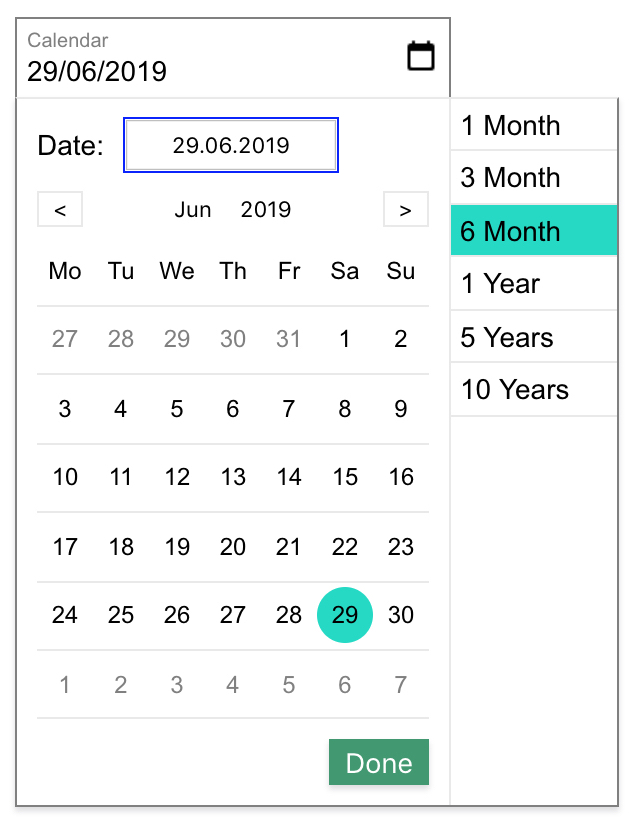The image depicts a digital calendar, likely from a mobile application, characterized by a sleek, modern design. A thin black line outlines the entire calendar, except for a small section with a gray border that protrudes slightly. In the upper left corner, the heading reads "Calendar 29/06/2019," accompanied by a black calendar icon in the upper right corner. Below, the text "Date:" is followed by a gray box with a blue outline, displaying "29.06.2019."

Navigation arrows flank the label "June 2019," allowing users to move between months. The calendar grid is organized into columns labeled Monday through Sunday, with rows indicating dates starting from the previous month's Monday, the 27th, and continuing through to the current month's Sunday, the 30th. Key dates are highlighted, with the 29th of June marked in blue.

At the bottom of the calendar, a prominent green button labeled "Done" appears in white text. To the right of the calendar, options for viewing different timeframes are listed: "One Month," "Three Months," "Six Months," "One Year," "Five Years," and "Ten Years," with "Six Months" currently selected.